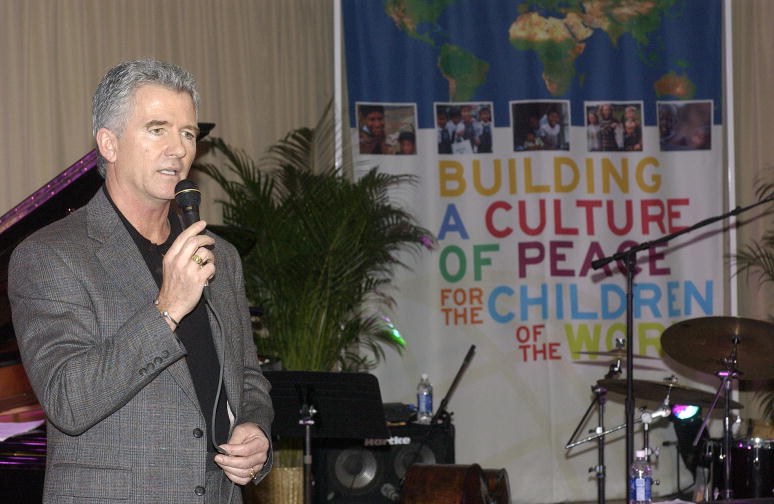On a warmly-lit stage set for a music event, a light brown curtain serves as the backdrop for an array of musical instruments. Hanging prominently is a banner featuring a world map, accompanied by five photographs of different individuals. Below these images, the banner proclaims: "Building a Culture of Peace for the Children of War." To the right of the stage, a drum set awaits its player. A large, verdant plant, elegantly fanned out, stands tall next to the banner, adding a touch of nature to the scene. Adjacent to the plant is an open-top purple piano, adding a splash of color to the setup. At the forefront of the image is a distinguished gentleman with gray hair, holding a microphone and addressing the audience. He is dressed in a gray suit paired with a black shirt, exuding an air of sophistication and calm authority.